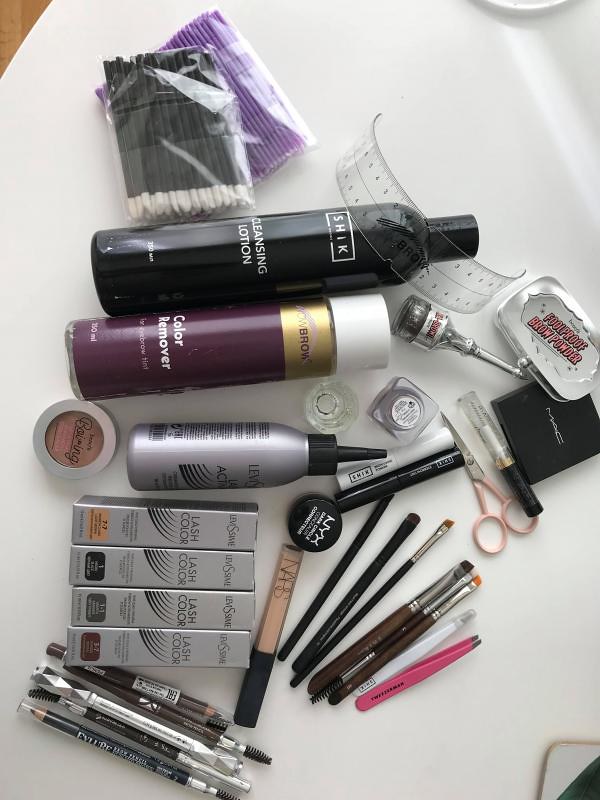In this image, we observe an extensive array of beauty items laid out meticulously. 

Starting from the left side, a set of tightly wrapped purple items, each about two inches in length, catches the eye. Above these, a collection of black eyeshadow applicators with white tips is prominently displayed. Moving right, a black bottle labeled "Cleansing Lotion" sits next to a color remover bottle, distinguished by its burgundy body and white cap. Both bottles partially obscure the image of the top half of a ruler.

Next, several Benefit makeup products are evident, including a brow powder and another brow product with a long silver tip. Nearby, a small black compact sits above a tiny pair of pink nail cutting scissors. Adjacent to these, a white tube and a black tube lie side by side.

To the right, small angled makeup brushes are aligned neatly. Directly beneath these brushes, a NARS container, presumably for concealer, is positioned. Below this, the layout features four silver boxes, which likely house different shades of eyeshadow, each adorned with images of eyelashes on their fronts. 

Finally, the collection includes what appear to be four eyeliners, featuring varying shades – some silver, others black, and one brown – completing the carefully curated assembly of beauty products.